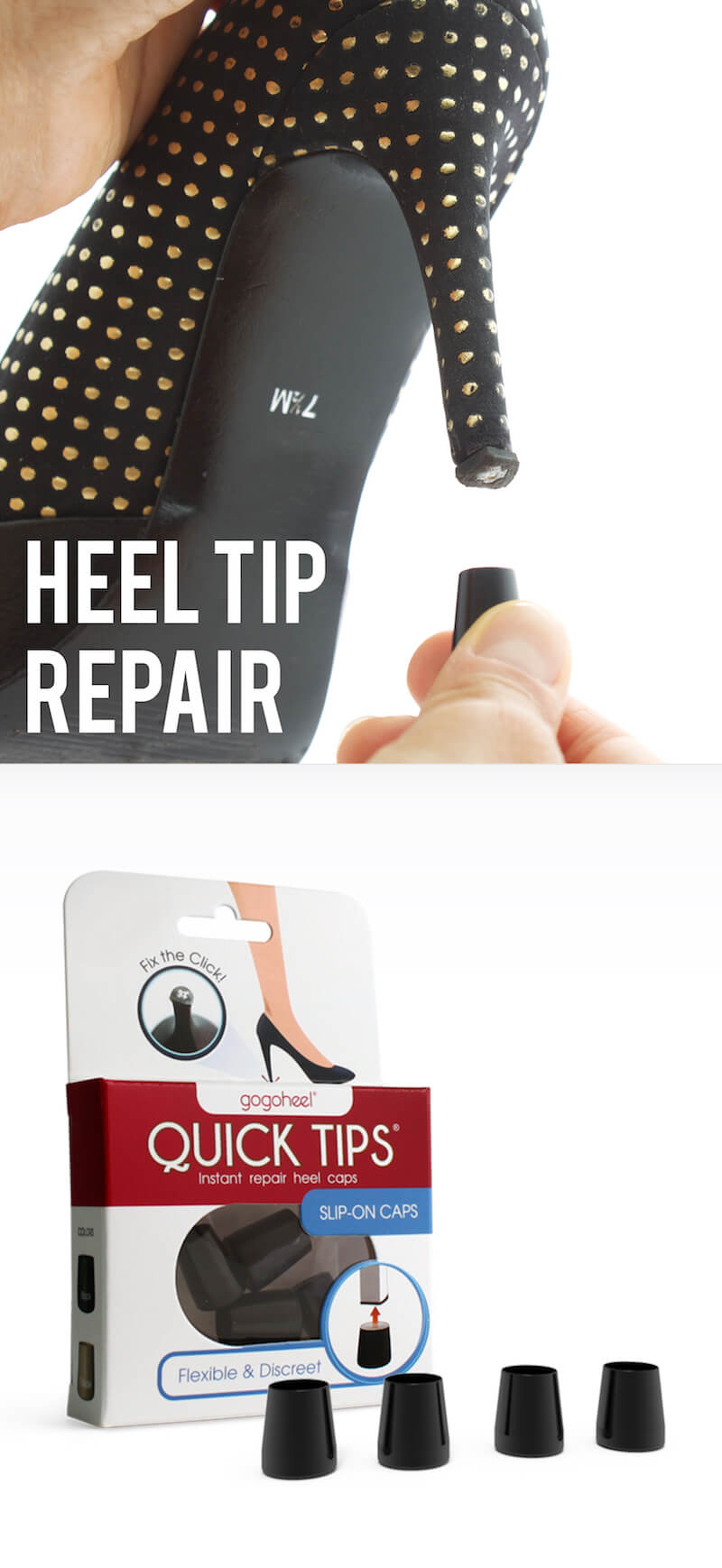The advertisement prominently features a product designed for heel tip repair. The upper section of the image showcases a close-up of a black high heel shoe adorned with small gold polka dots. A left hand holds the shoe while a right hand is poised to attach a new heel tip, emphasizing the repair process. Bold white text in the bottom left corner of this section reads, "Heel Tip Repair." 

The lower section of the image displays the product packaging and its contents against a clean white background. The packaging, branded as "Go Go Heel," prominently features the text "Quick Tips" in red. Below this, the phrases "Slip on Caps," "Flexible and Discreet," and "Fix the Click" highlight the product features. The packaging includes an illustration of a leg wearing a high heel shoe, with an arrow indicating how the slip-on caps should be applied. Four example heel tips are arranged in front of the box, illustrating the components included for instant heel repairs. The overall design conveys the ease and convenience of using the heel repair caps to eliminate the clicking sound and extend the life of high heel shoes.